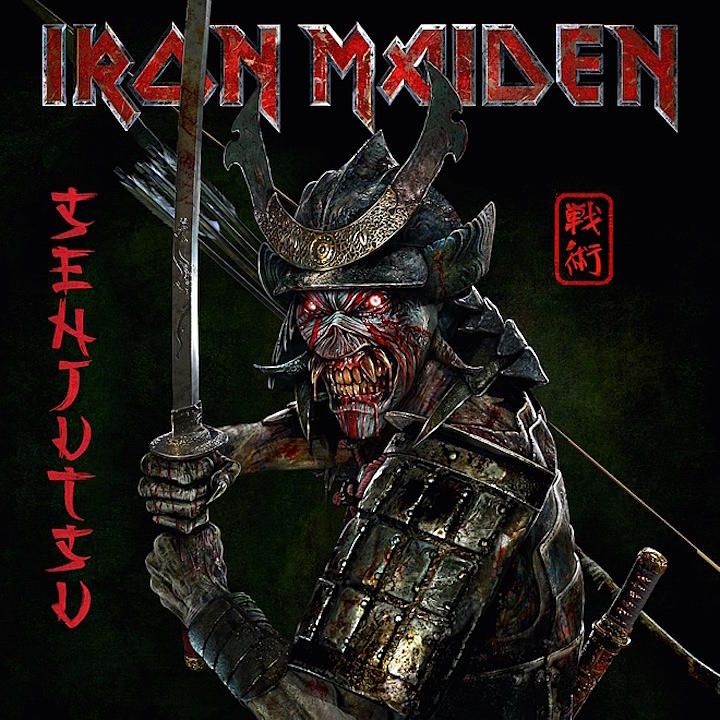This image is a square poster, measuring approximately 6 inches by 6 inches, featuring a predominantly black background. At the top, the title "Iron Maiden" is prominently displayed in bright red, blood-like letters with a silver metallic beveled edge. 

Dominating the center of the poster, there is a formidable creature. From the waist up, the figure resembles a zombie outfitted in an armored samurai uniform. The creature's menacing face, reminiscent of a zombie monkey, showcases large fangs and glowing red eyes that ooze blood, enhancing its terrifying appearance. Its half skeletal, half metal visage is crowned with a Viking-style helmet. 

The creature wields a sword in its hands, angled towards the left side of the poster. Over its back, several arrows protrude from a quiver, indicating readiness for battle. Additionally, a baton-like object can be seen sticking out on the right. 

Flanking this central figure, on the left side of the poster, are vertical red letters resembling Japanese kanji. Similarly, on the right side, a red-bordered rectangle encloses more red Asian-style script. These elements further contextualize the dark, combat-ready theme of the image, with subtle green smudging around the figure adding depth to the stark black background.